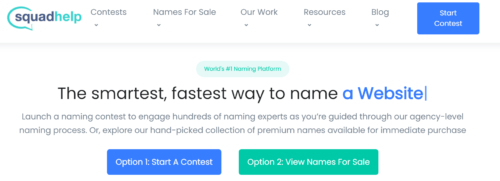The website depicted is called "Squad Help." The word "Squad" is in navy blue, while "Help" is in turquoise. The logo features a half-circle resembling the letter "C" over the letters "S-Q-U." Below the logo, there are several clickable gray buttons labeled "Contests," "Names for Sale," "Our Work," "Resources," and "Blog," each accompanied by a small arrow.

To the far right, a blue banner displays the text "Start Contest." Beneath it, a green banner proclaims "world's number one naming platform" in green letters. Below this banner, a black text block reads "the smartest, fastest way to name a website," with "A Website" highlighted in blue. Further down, in gray text, the website states: "Launch a Naming Contest to Engage Hundreds of Naming Experts as You're Guided Through Our Agency Level Naming Process, or Explore Our Handpicked Collection of Premium Names Available for Immediate Purchase."

At the bottom, two prominent banners offer options. A blue banner with white text reads "Option 1: Start a Contest," while a green banner with white text reads "Option 2: View Names for Sale." These banners likely serve as interactive buttons for users to either start a naming contest or browse available premium names.